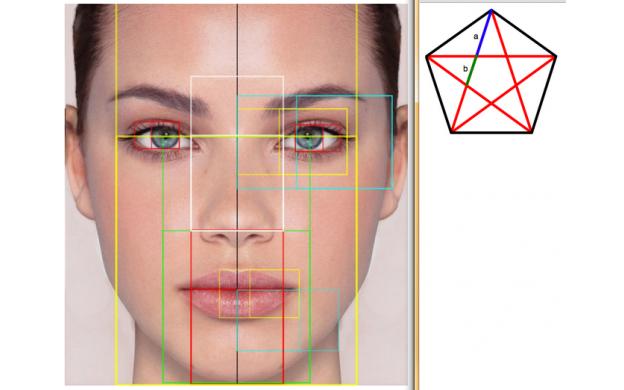This image presents an up-close schematic of a woman's face, spanning from her chin to the top of her forehead, with her ears and a sliver of black hair visible. The woman has dark brown eyebrows, striking blue eyes with pink eyeshadow, and soft pink lips. Overlaid on her face are several colored lines and geometric shapes used for facial analysis:

- Two vertical yellow lines outline the edges of her face, from her eyebrows to her chin.
- A black vertical line runs down the center of her face, bisecting her nose and lips.
- A horizontal yellow line crosses her face through the middle of her eyes.
- A white box encases the width of her nose, extending from her lower forehead to the area between her eyes.
- Two red lines drop from the white box to the nearly reach the corners of her lips.
- A small yellow box frames three-quarters of her right lips.

To the right side of the image is a detailed five-sided figure (pentagon) containing a red star. Segments within the star are highlighted with blue and green sections, labeled 'A' and 'B' respectively. This diagram likely aims to illustrate the symmetry and ideal proportions of the face, suggesting a mathematical or aesthetic analysis of beauty. Overall, the image combines artistic and scientific elements to assess facial symmetry and harmony.